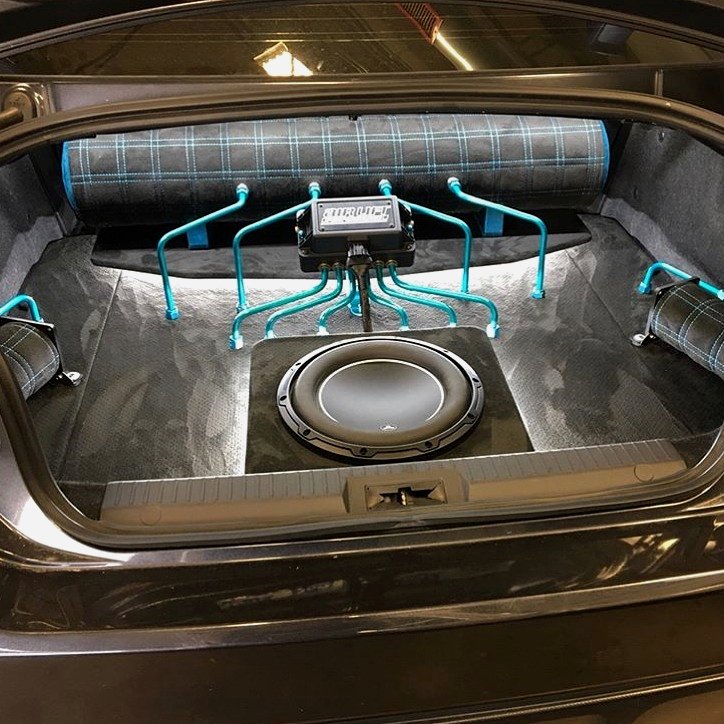Inside the trunk of the vehicle, the interior is a dark gray color, which seems to have been modified. There's a round speaker installed, connected to blue metal cords that run from the bottom of the trunk. These cords lead to a structure that appears to be wrapped in a cloth-like material, resembling a blanket but likely serving a different purpose. This protective covering is predominantly gray with a plaid pattern, featuring both horizontal and vertical striped lines. The cloth is encased within a metal tube, adding to its unusual appearance.